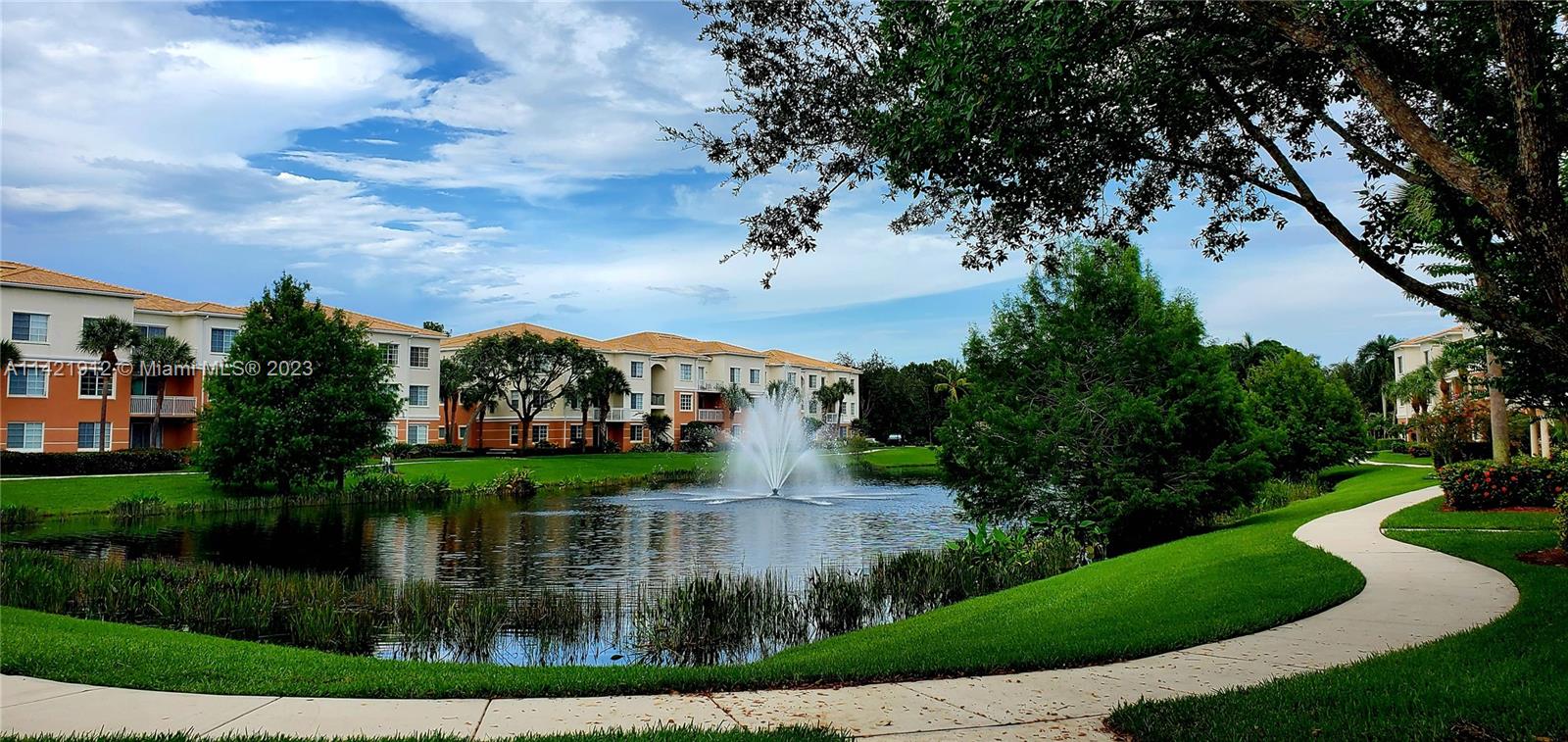The landscape photo is an elongated, rectangular image showcasing a tranquil outdoor setting, likely a suburban area in Miami, as indicated by a small watermark reading "Miami ALS, copyright 2023." Dominating the center of the photograph is a large pond featuring a water fountain that creates gentle ripples. Surrounding the pond is a well-manicured lawn, lush green grass, and a concrete pathway that curves gracefully, encircling the water. The foreground displays a mixture of grass, trees, and flowering bushes, adding to the picturesque scene. In the background, under a blue sky dotted with a few wispy clouds, stands a three-story apartment building. The building features burnt umber coloring for the first two stories and a whitish hue for the top story, topped off with orange roofs. This peaceful depiction of real life captures a serene housing development, potentially on a golf course, and evokes the charm of a sunny day in central Florida.